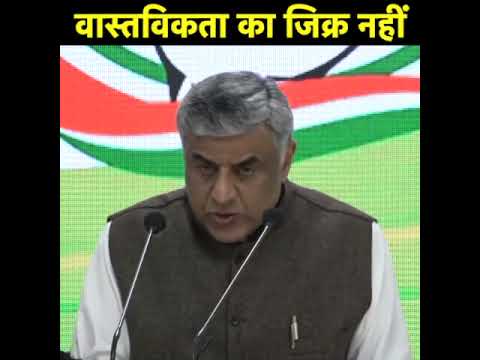The image depicts an older Eastern Indian gentleman, likely in his late 50s, speaking into two small black ball-shaped microphones positioned on a white stand. He has a salt-and-pepper complexion with short, gray and black hair lying flat on his head. He is dressed in a brown suede vest adorned with a pin, over a long-sleeve white shirt. His mouth is slightly open, indicating he is in mid-speech.

The backdrop is visually distinctive, featuring a projector display with several wavy color patterns. The bottom portion is light green, topped by a wave of dark green and then a flipped version of this wave in red. The spaces in between these waves are white, while above them sits another green wave. Around the gentleman, a black outline provides contrast to the background. Above him is text in yellow, composed of Asian characters, likely Middle Eastern or Indian, connected by dashed lines with words extending downward. The overall scene suggests a formal setting, possibly a significant address or speech.